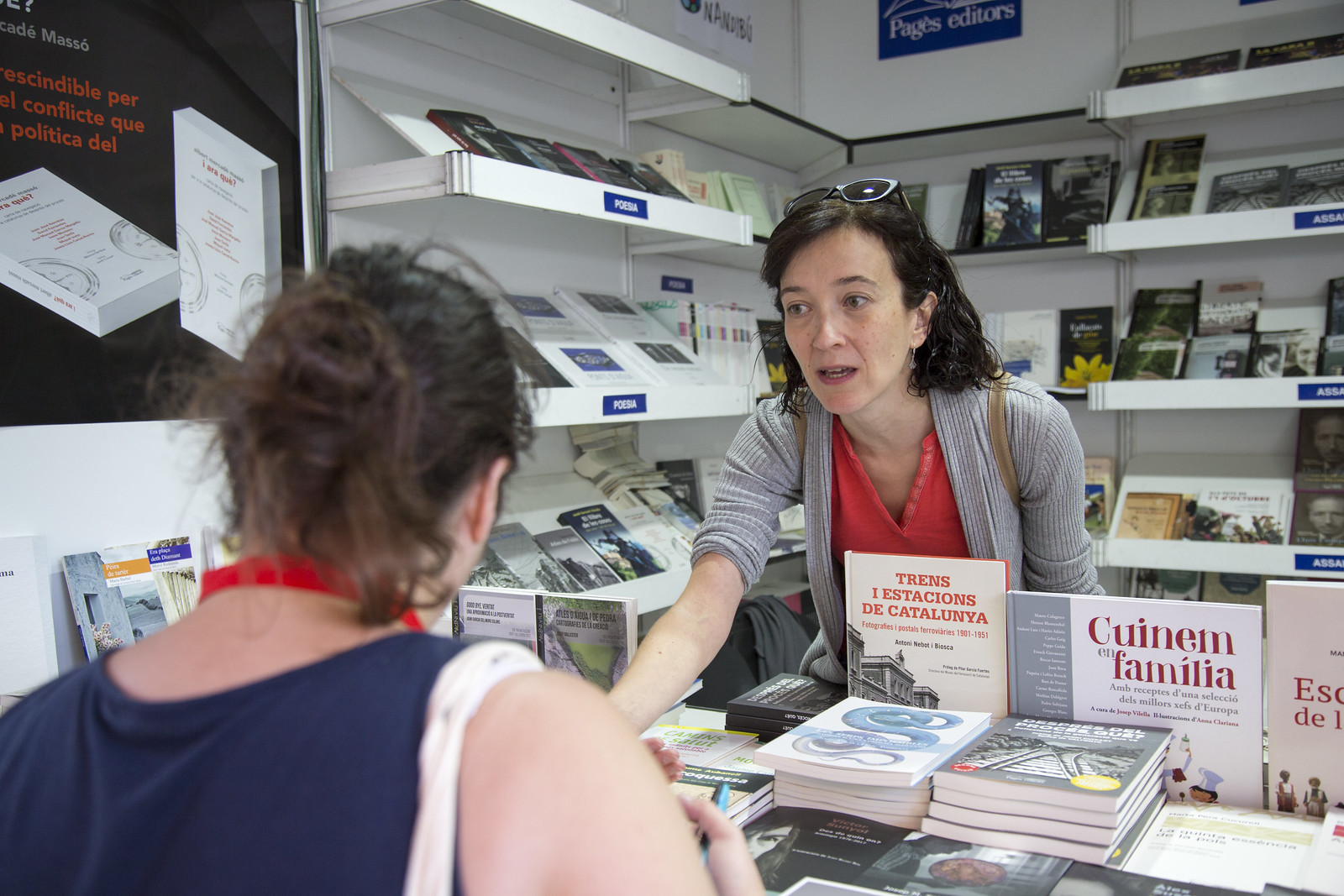The image captures a lively scene at a bookstore or book exhibit, featuring two women engaged in conversation over a table densely packed with books. The woman behind the table has dark hair and is dressed in a gray cardigan layered over a red V-neck top. She also has sunglasses with blue frames perched on her head. Books with titles in Spanish such as "Trends," "Estaciones de Cataluña," and "Unión de Familia" are prominently displayed on the table. In the background, shelves filled with more books create a busy backdrop. The woman facing the camera, in a blue tank top with a red lanyard around her neck, has her hair tied in a ponytail and seems to be inquiring about a book or perhaps making a purchase. The scene is rich with literary ambiance, underpinned by the visual clutter of numerous books in various colors and languages.